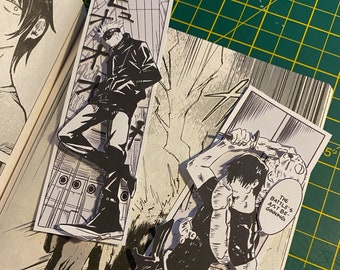A black-and-white comic book is opened on a uniquely patterned table displaying a green and yellow square design. The comic book, laid out at a slight angle to the right, extends beyond the left side of the image, cutting off a portion of the pages. Enhancing the scene, a bookmark that features artwork matching the style of the comic book is tucked between its pages. The table's vibrant colors contrast with the monochrome comic, setting the stage for a vibrant tableau.